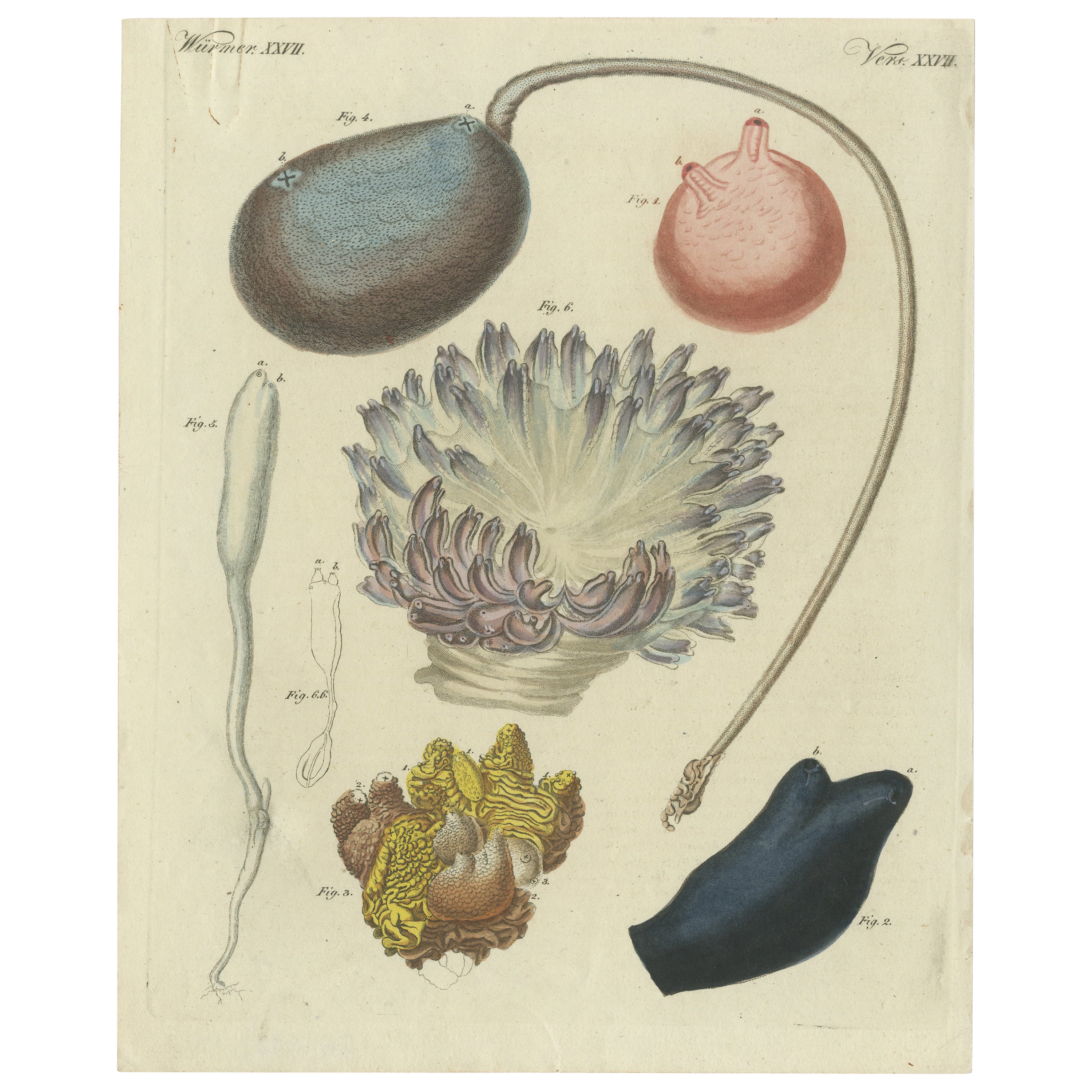This image appears to be a detailed diagram from a book, possibly showcasing various biological or botanical sketches. In the top left corner, it is labeled "Vormer XXVII," while the top right corner is marked "Vena XXVIII." The diagram consists of six distinct drawings, each identified by figure numbers. 

- The top left drawing (Figure ?) depicts a gray circle with a prominent tube extending from it.
- The top right drawing (Figure ?) shows a pink circle with several small nubs protruding from its surface.
- Among the other figures is an oval-shaped, brown to black object (Figure 4?) with a long, curved stem.
- Another notable figure resembles a long, white cottontail, possibly identified as Figure 4 in different listings.

Additional details include a light red object, a gray-black item, a black oblong shape at the bottom right, and a yellow blob in the bottom center. The items depicted might represent different creatures or close-ups of plant parts.